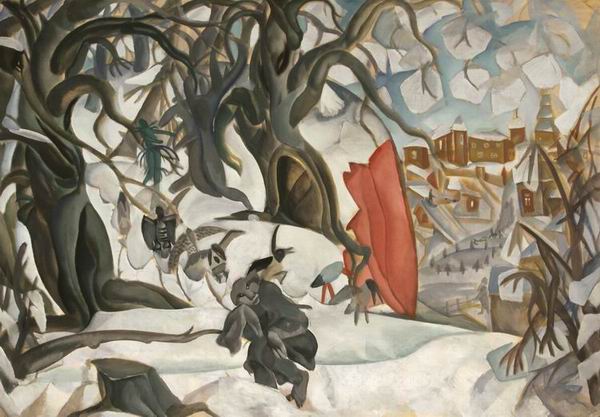In this somewhat abstract, yet slightly representational painting, the artist depicts a fantastical outdoor winter scene during the daytime. The foreground is dominated by a blanket of snow and stark, leafless, dark trees with long, wavy branches that seem almost enchanted or spooky. Among the snow-covered ground, a series of birds, possibly pigeons or ducks, are standing. There is also a lone figure dressed in a black or gray outfit, head obscured, walking through the snow. Further to the left, a creature resembling reindeer or horned horses adds to the fantastical element.

The background reveals a road leading towards a village with several buildings, including houses with lights on, and a prominent two-story building with gabled roofs. Beyond that, a multi-storied tower tapers upwards, enhancing the imaginative atmosphere. 

The sky is rendered in shades of gray and light blue, with shapes reminiscent of cotton, contributing to the surreal quality of the scene. Additional details, like a red hill or cliff towards the center and snow stuck to the branches in the top-right of the painting, further enrich the composition. The overall effect is a dreamlike winter landscape that straddles the line between reality and fantasy.